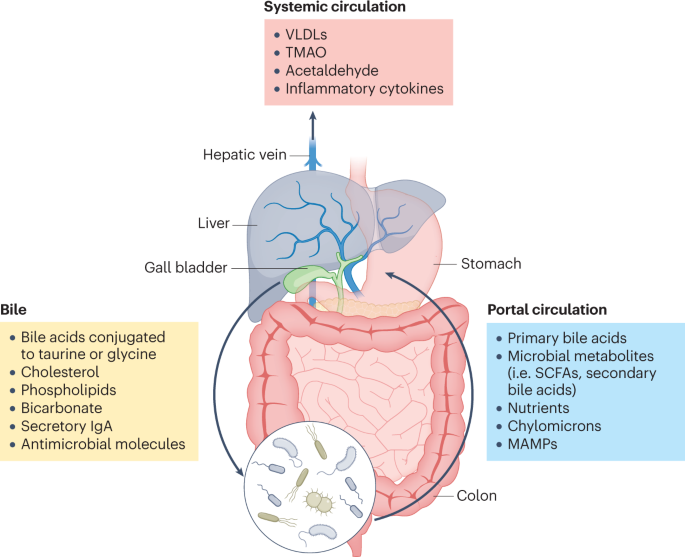The image is a digital slide from an educational presentation on the digestive system and related circulatory pathways, set against a white and black background. At the top, it is labeled "Systemic Circulation" followed by a pink rectangle with bulleted points reading "VLDLs, TMAO, acetaldehyde, inflammatory cytokines."

Central to the diagram is a detailed illustration of the digestive system showing the liver, stomach, gallbladder, intestines, and colon in distinct colors with black labels. The stomach, highlighted in pink, contains a zoomed-in section showing bacteria. To the left, the diagram includes the hepatic vein and bile components detailed in a yellow rectangle. Key terms associated with bile such as bile acids conjugated to taurine and glycine, cholesterol, phospholipids, bicarbonate, secretory IgA, and antimicrobial molecules are listed.

On the right, the diagram describes portal circulation in a blue box, mentioning additional terms such as SCFS, primary and secondary bile acids, chylomicrons, MAMPs, and microbial metabolites. The overall setup conveys essential details of digestive and hepatic processes with extensive annotations and vivid color coding.